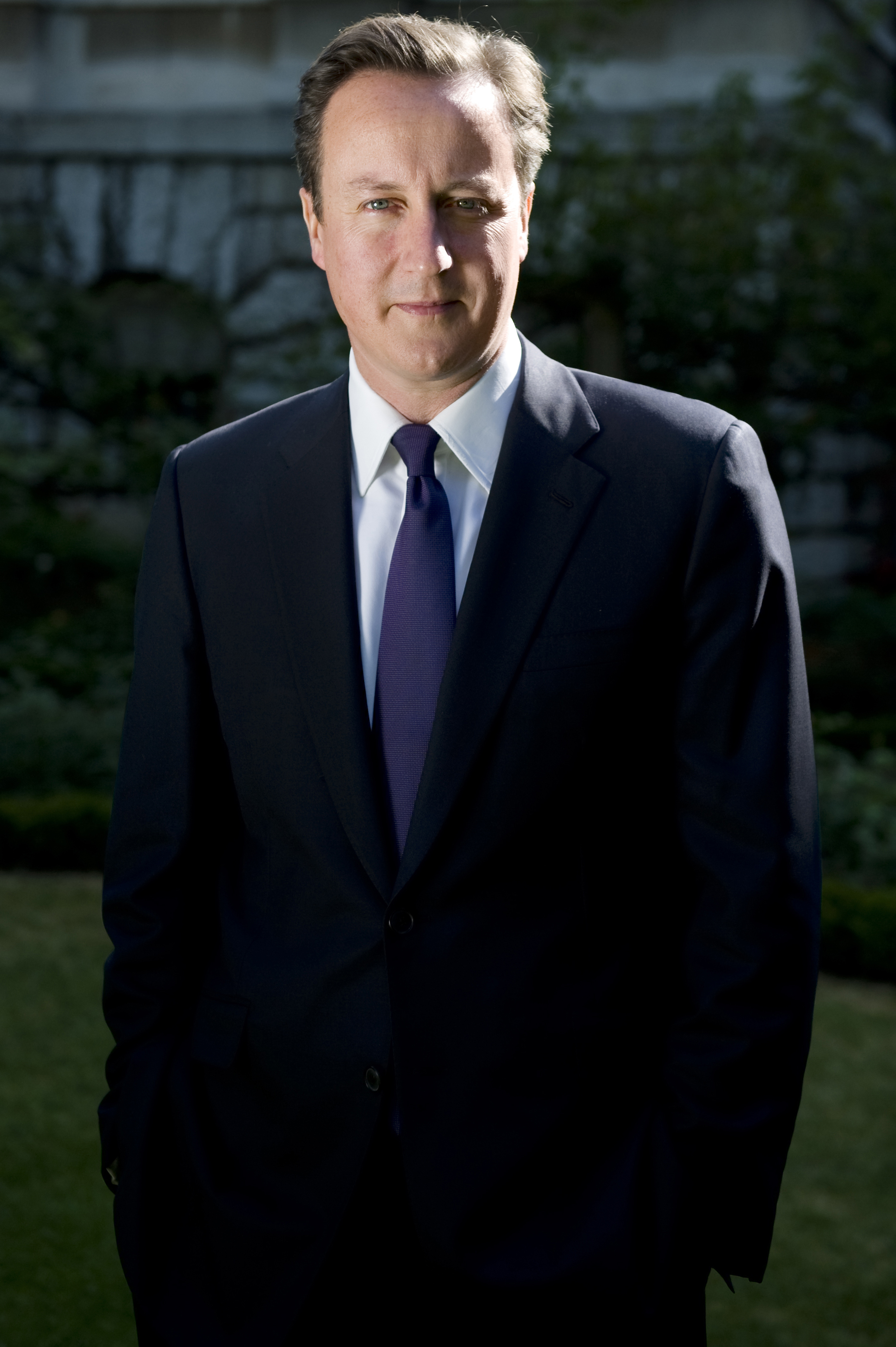In this photograph, a Caucasian man with greenish-gray eyes is looking directly into the camera. He's dressed in a dark suit, a white shirt, and a purplish-blue tie, with his hair combed back. Standing very tall with broad shoulders and a wide torso, he has his hands in his pockets and exudes a slightly serious demeanor, softened by a faint smile. The early morning sun casts light on his shoulder and face, creating a striking contrast of bright sunlight and shadows. Behind him, a yard with green grass leads to various plants and shrubbery, with small trees marking the boundary. Further back, a stone building, resembling a house, stands prominently, flanked by bushes.